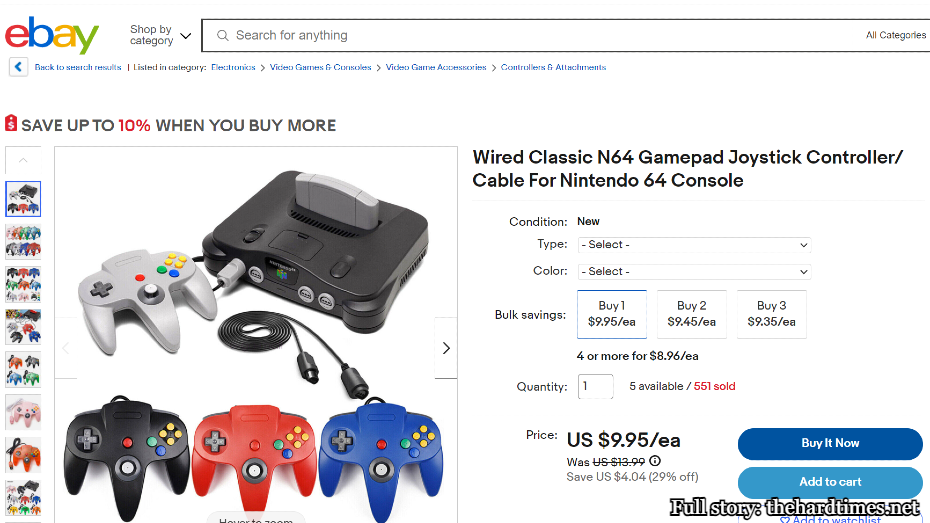The image showcases an eBay webpage. In the top left corner, the iconic "eBay" logo is prominently displayed with the letters in different colors: 'e' is red, 'b' is blue, 'a' is yellow, and 'y' is green. At the top of the page, there are navigation options including "Shop by Category" and a search bar with the placeholder text "Search for anything."

Beneath the eBay logo, tabs provide navigation paths such as "Back to Search Result," "Listed in," and categories including "Electronics," "Video Game & Console," "Video Game Accessories," "Controller & Attachments."

On the left side of the page, there is a promotional message: "Save up to 10% when you buy more," with the "10%" highlighted in red and the rest of the text in black.

The main product showcased is a device with several controllers displayed in different colors: a grey one, a black one, a red one, and a blue one. Additional images of controllers in various colors are also displayed on the left side of the page.

To the right of the product images is a detailed description of the item: a wired classic N64 controller compatible with Nintendo 64. The condition of the product is marked as "New," and there are options to select the type and color of the controller. 

The pricing breakdown reveals bulk savings: 
- Buy one for $9.95 each
- Buy two for $9.45 each
- Buy three for $9.35 each
- Four or more for $8.90 each

Currently, a quantity of one is selected, with five units available in stock marked in red.

The previous price of the item was $13.99, but it is now offered at $9.95 each, noting a saving of $4.04, which is 29% off.

At the bottom right, two buttons for purchasing options are displayed: "Buy It Now" in blue, and "Add to Cart" in light blue. 

Finally, at the bottom of the page, there is a message that reads: "Full story: dhardtimes.net."